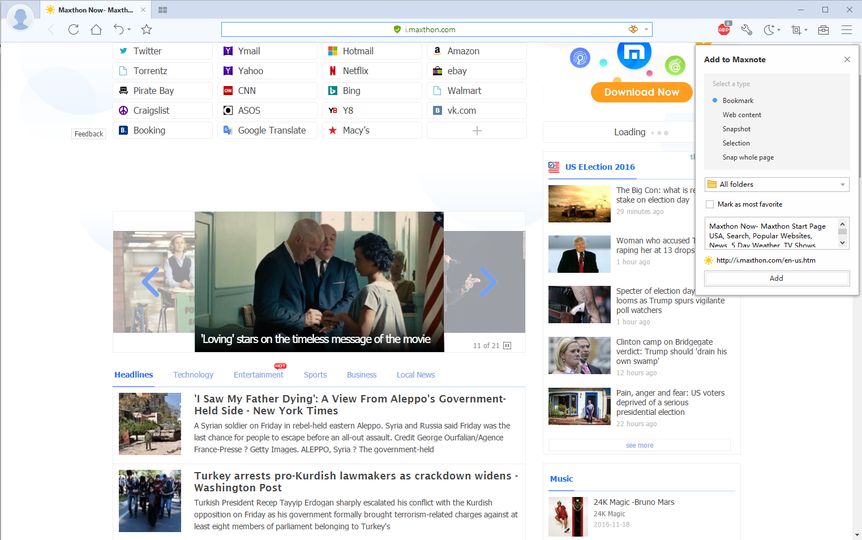This screenshot captures an unknown website, notably featuring the Maxthon browser. The address bar reads i.maxthon.com. At the top section, a menu displays several well-known websites: Twitter, Torrance, Pirate Bay, Craigslist, Booking, My Mail, Yahoo, CNN, ASOS, Google Translate, Hotmail, Netflix, Bing, Y8, Macy's, Amazon, eBay, Walmart, and VK.com.

Central to the page is an image depicting three people in what appears to be a courtroom setting, captioned with "Loving stars on the timeless message of the movie." Below the image, a navigation bar lists categories such as Headlines, Technology, Entertainment, Sports, Business, and Local News, with "Headlines" being selected.

Highlighted news stories include:
1. "I saw my father dying, a view from Aleppo's government-held side" (New York Times), describing a Syrian soldier in rebel-held eastern Aleppo, with an urgent message from Syria and Russia about the final chance for people to escape before a major assault. The photo credit is given to George Orfolian/Agence France-Presse/Getty Images, Aleppo, Syria.
2. "Turkey arrests pro-Kurdish lawmakers as crackdown widens" (Washington Post), detailing Turkish President Recep Tayyip Erdogan's aggressive actions against the Kurdish opposition, including terrorism-related charges against members of parliament. The article is cut off at this point.

On the right side of the screen, there is a vertical drop-down menu featuring options such as Add to Max Note, Bookmark, Web Content, Snapshot, Selection, Snap Whole Page, along with several navigation folders and settings like Mark as Most Favorite, Maxthon Now, and Maxthon Start Page. This menu also includes several sections focused on USA, Search Popular Websites, News, Five-Day Weather, TV Shows, and U.S. Election 2016. Some headlines are partially obscured by this drop-down menu, including: "Clinton camp on Bridgegate verdict, Trump should drain his own swamp," "Pain, anger, and fear: U.S. voters deprived of a serious presidential election," and a music headline about "24K Magic" by Bruno Mars.